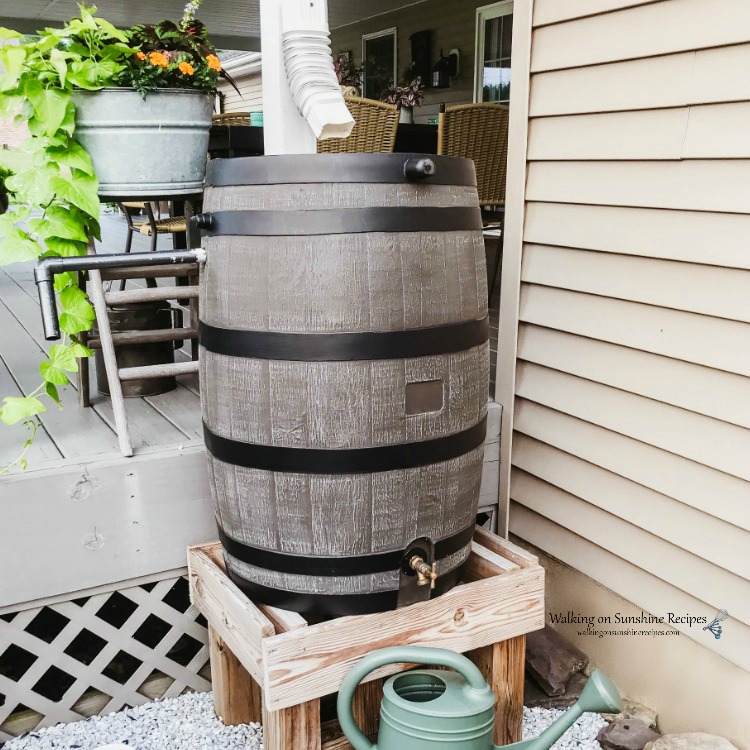In the middle of this square, daytime photograph taken outdoors in someone's backyard, you see a light gray rain barrel with black horizontal lines. The barrel sits on a brown wooden stool with a non-flat top. The barrel features several components, including a pipe sticking out from its left side and a gold spigot at the bottom. A hose can be seen coming from the roof, leading into the barrel, suggesting it's part of a rainwater collection system. Directly under the spigot on the ground, there's a green plastic watering can without a lid. In the background, there's a mix of arrangements, with the beige horizontal siding of the house visible on the right and a gray-painted wooden deck area on the left that holds a metal bucket with green ivy plants. To the right of the barrel, black lettering reads "Walking on Sunshine Recipes," and beneath that, "WalkingOnSunshineRecipes.com."